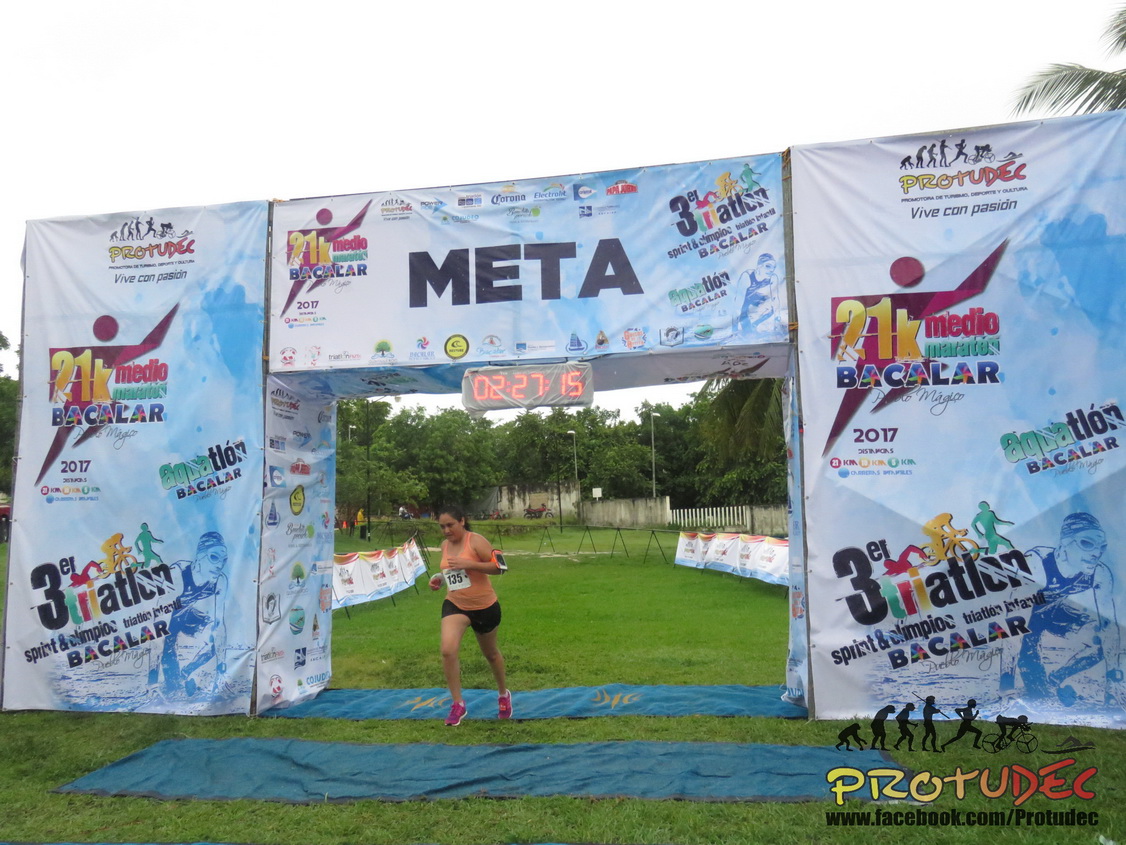The photograph captures a woman running through a rectangular archway in a grassy field, likely the finish line of a race. The archway, constructed with two columns and a connecting horizontal beam, is adorned with canvas-style banners featuring various advertisements, radio station logos, and the word "META." A digital sign hangs from the horizontal beam, displaying the time "02:27:15" in red text. The runner, identifiable by her peach tank top, dark shorts, and bright pink sneakers, has her knees bent in mid-stride and wears a race number on her front. Additional text on the banners includes "3ER triathlon." The scene suggests a competitive event, possibly a 21k race, occurring in 2017.